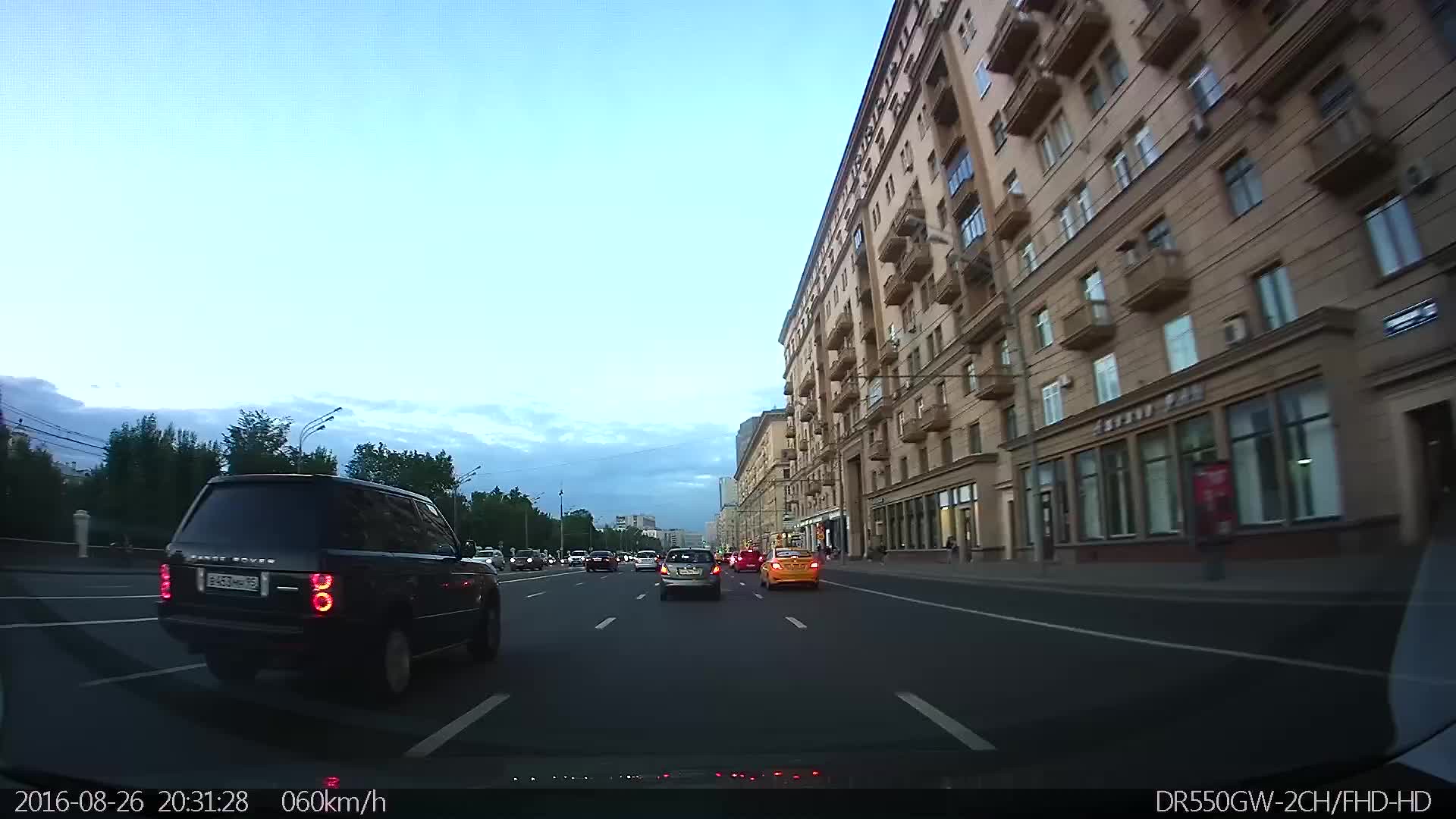This image, taken from inside a moving vehicle, captures a bustling street scene on August 26th, 2016, at 20:31:28 (military time). In the lower left-hand corner, a street cam timestamp is visible. Centered on the street, white lines delineate the traffic lanes. Close in, a black SUV truck is directly ahead of the capturing vehicle. To the SUV's left, a gray car is braking, its brake lights glowing red. In the adjacent right lane, a yellow vehicle is visible, followed by a red car ahead of it.